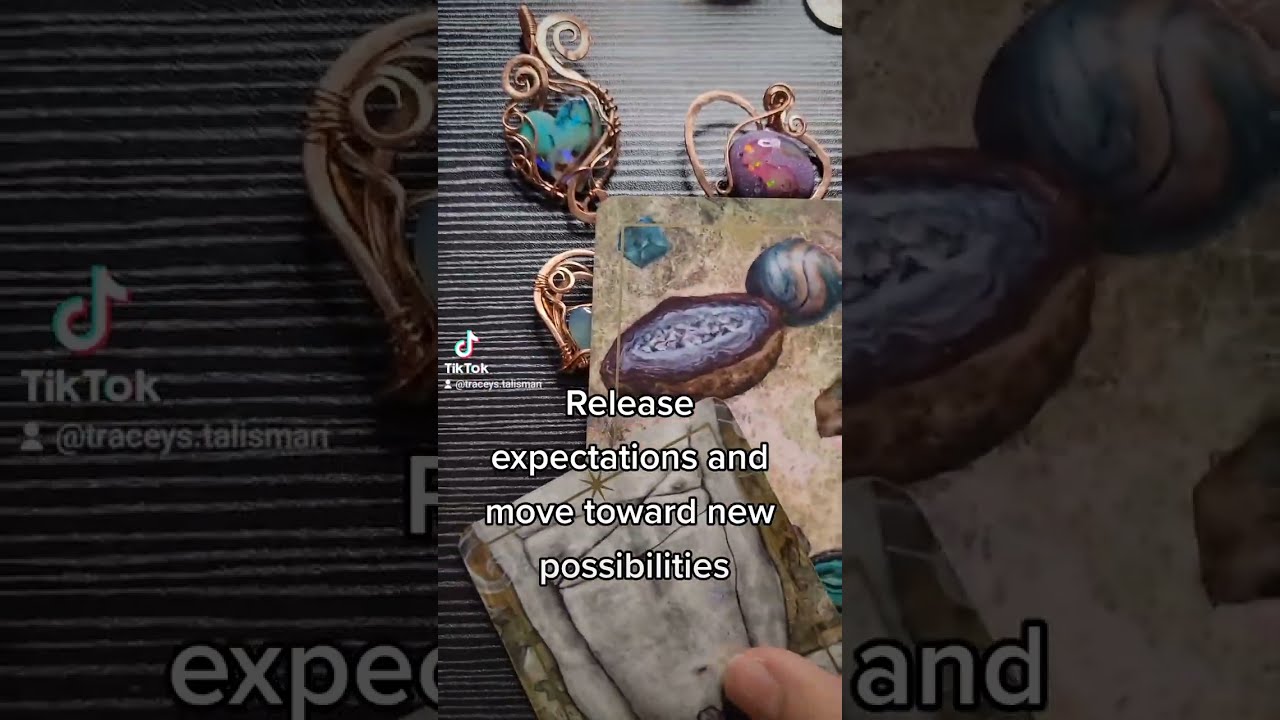The image is a detailed and vibrant vertical landscape, segmented into three parts—a bright, central image flanked by darker, zoomed-in portions of the same picture on the left and right. The focal point is a textured, wood-like table surface adorned with intricate, decorative objects. Prominently displayed near the bottom center is a motivational text in white lettering that reads, "Release expectations, move toward new possibilities," spanning four lines. The top left corner features the recognizable TikTok logo.

On the table surface, various gemstones in shades of purple, teal, and aqua, and other colors, are placed. These gems are encircled by whimsical, gold squiggly designs, resembling pendants and other pieces of jewelry, including beautifully wrapped little crystals. There also appears to be a hand holding a small, rectangular piece towards the bottom right, adding a layer of interaction to the scene. This piece may be a card, with a noticeable brown border against a primarily gray background. Overall, the arrangement of vibrant gemstones, intricate jewelry, and motivational text creates a rich, inspiring visual tapestry.